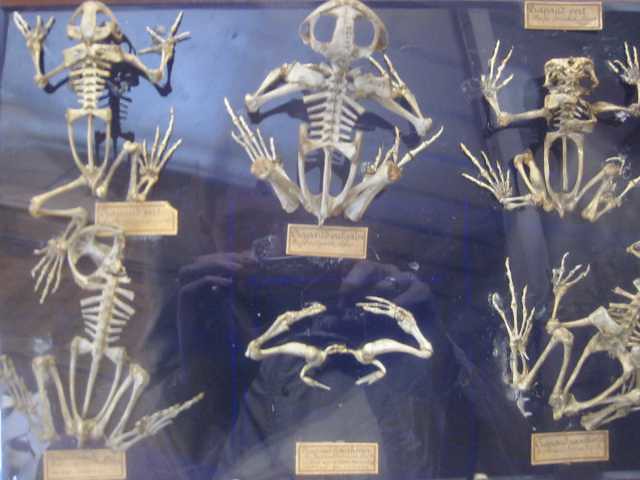The image shows a collection of small animal skeletons, likely frog skeletons, displayed in a glass case mounted against a blue background. There are six skeletons arranged in two rows, with three per row. Each skeleton is fixed on a small brown mount. Notably, the skeleton positioned at the bottom center is incomplete, displaying primarily leg or hand bones. Small identification tags accompany each skeleton, but they are too small to be legible. The tag for the skeleton in the top right corner is uniquely placed above rather than below. A person, identifiable by their reflection in the glass, is capturing the image. They are wearing long sleeves and a ring on their left hand.